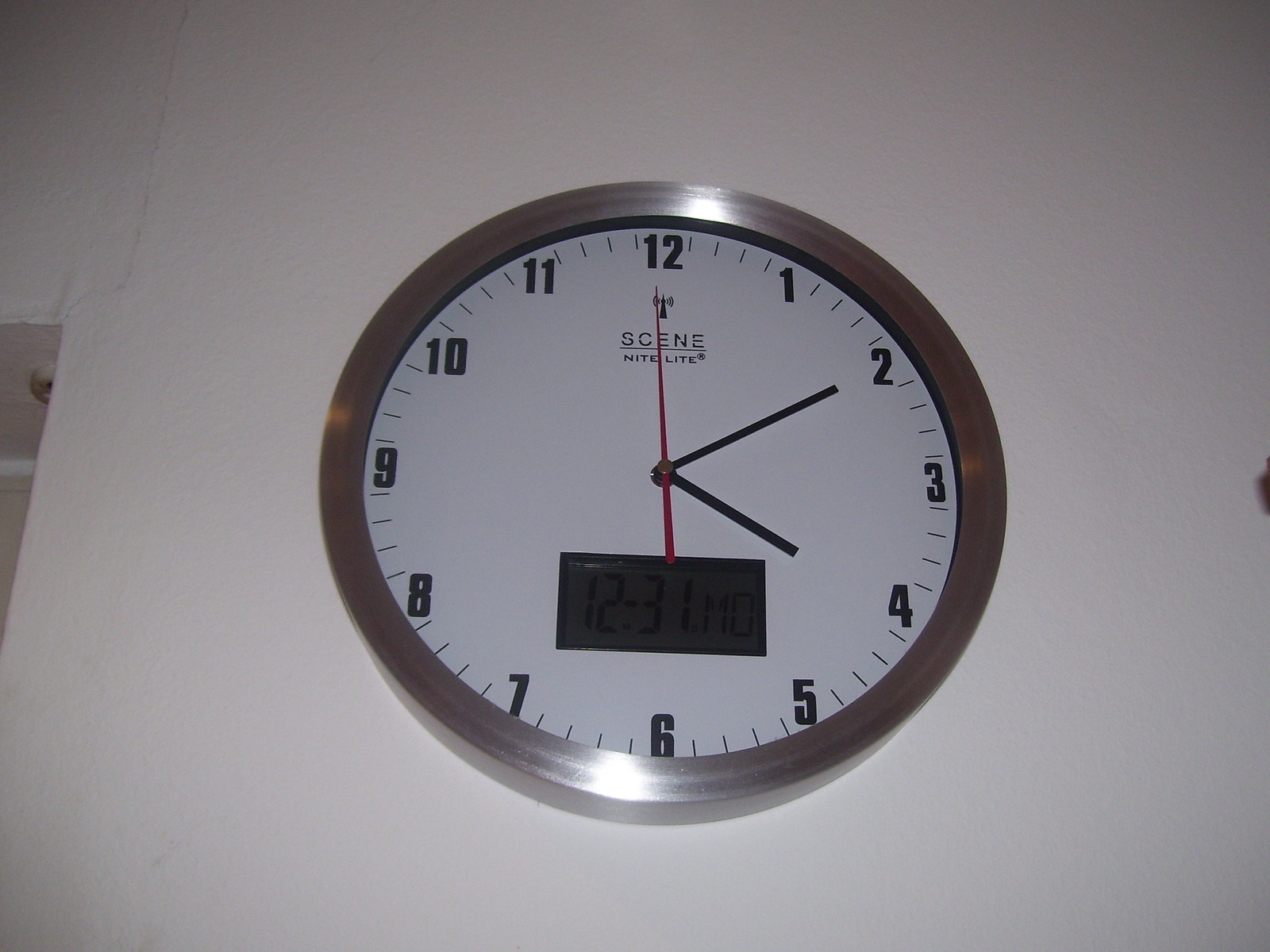This color photograph captures a round clock mounted on a pristine white wall. The clock features a sleek silver outer casing and a glass cover protecting its face. The face of the clock is crisp white, adorned with bold black numbers and matching black hour and minute hands. A vibrant red second hand adds a touch of contrast, making the time easily readable. At the top, just beneath the 12 o'clock mark, the manufacturer's logo is prominently displayed, reading "SceneNiteLite." Situated above the 6 o'clock position is a digital display, clearly showing "12:31 MO." The photograph is devoid of any people, animals, plants, flowers, or trees, focusing solely on the clock against its simple backdrop.